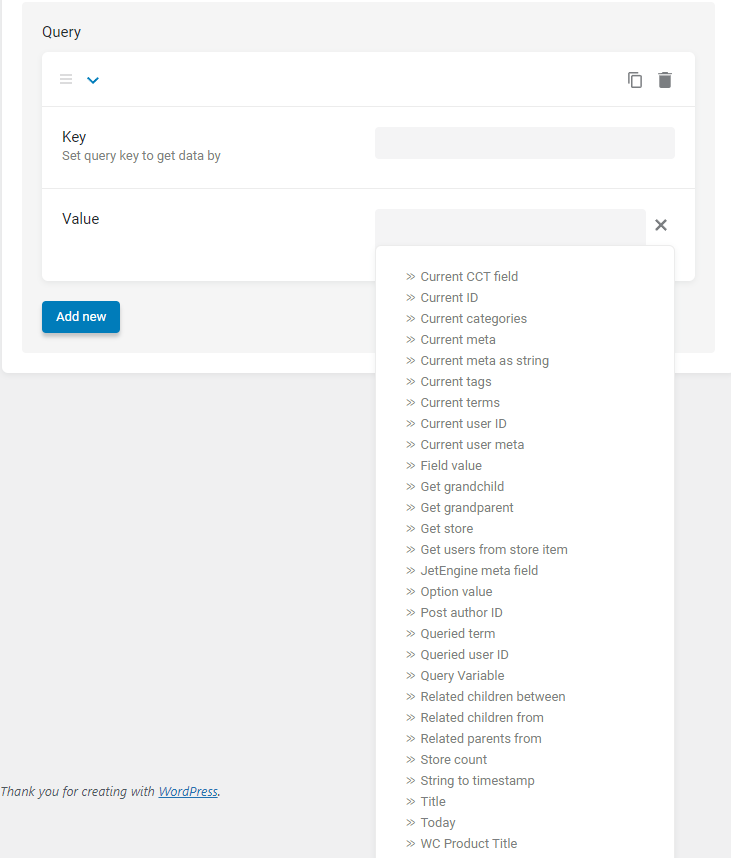A detailed interface screenshot showcases a query construction site. The upper left corner features a drop-down menu labeled "Queries," enabling users to select different query options. On the upper right, icons resembling a trash can and a possible duplication symbol are visible, although the latter is not explicitly labeled. 

Beneath these icons, there's a field titled "Key Field," with instructions indicating "set query key to get data back or data by." Adjacent to this field is a gray area, presumably for input or display purposes. 

Further down, a "Value Name" field is shown, accompanied by an extensive drop-down list of potential values on the right. Options in this list include:

- current CCT field
- current ID
- current categories
- current meta
- current meta a string
- current tags
- current terms
- current user ID
- current user meta
- field value
- get grandchild
- get grandparent
- get store
- get users from store item
- jet engine meta field
- option value
- post author ID
- query term
- queried user ID
- query variable
- related children between
- related children from
- related parents from
- store count
- string to timestamp
- title today
- WC product title.

On the bottom left, a note reads "Thank you for creating with," followed by a hyperlinked text in blue that directs to WordPress.